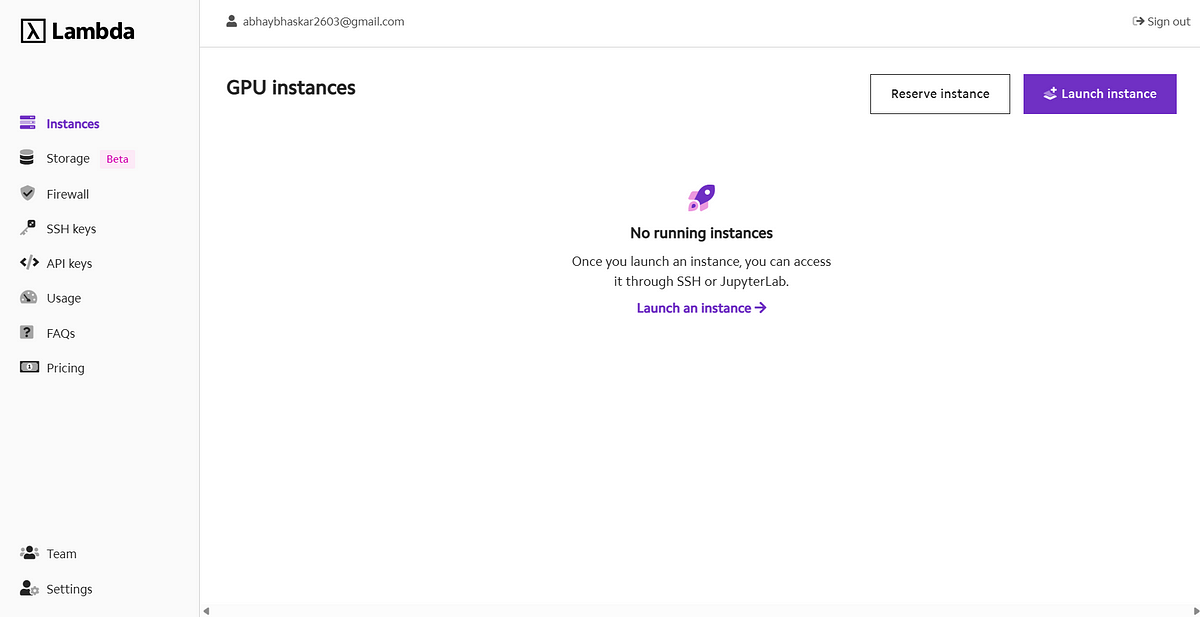Certainly!

---

The webpage for “Lombarda” features its logo on the top left, consisting of a black square with a teeter-totter symbol on the left. Adjacent to the logo is the company’s name. Below this, there's a cascading menu of options:

1. **Instances** - displayed in purple text.
2. **Storage** - represented by a stacked icon resembling pancakes, with an accompanying pink rectangle labeled "Beta" in hot pink text.
3. **Firewall** - illustrated with a dark gray shield bearing a black checkmark.
4. **SSH Keys** - depicted by a key icon.
5. **API Keys** - shown with greater than and less than symbols enclosing a backslash.
6. **Usage** - symbolized by a speedometer icon.
7. **FAQs** - accompanied by a gray box with a question mark.
8. **Pricing** - marked by a dollar icon.
9. **Team** - represented by a silhouette of three people.
10. **Settings** - shown by a single person silhouette with a gear icon.

In the central white area, a purple rocket ship with pink fins and pink flames is prominently displayed. Below this, bold black text states "No running instances." Further details in regular black text explain that users can access launched instances via SSH or JupyterLab. A hyperlink to "Launch an instance," styled in purple hypertext, leads users with a right-pointing arrow.

At the top left of the white area is a thin gray line in front of which is the user’s silhouette icon with the email "abhaybhaskar2603@gmail.com." To the right, text options include "Sign Out." Further down on the right side, bold black text reads "GPU Instances." Below this, two buttons are present: one white with "Reserve Instance" in black text, and another purple button labeled "Launch Instance" in white text, featuring a gray square on top of a white square with a plus sign.

---